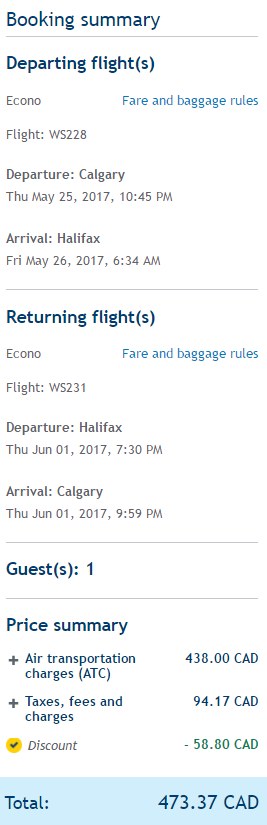A detailed screen capture, presumably from a cell phone, displays a booking summary from a travel website. The interface features flight information against a white background with a greenish-gray bold font. At the top left corner, "Booking Summary" is prominently displayed. Below it, separated by a gray line, the "Departing Flights" section is visible. In this section, gray lettering details the departure as "ACANO, Flight" from Calgary, along with the departure date, and the arrival in Halifax, including the arrival date. The upper right-hand corner of this section is marked with green lettering that reads "Fare and Baggage Rules."

A subsequent section, also separated by a gray line, is labeled "Returning Flights" in bold greenish-gray font. On the left, it specifies "ACANO, Flight" departing from Halifax and the departure date, arriving in Calgary on the specified date. On the upper right, "Fare and Baggage Rules" is again highlighted in light green.

The remainder of the page showcases details in the same bold, dark grayish-green font. It states "Guests: 1" and under "Price Summary," distinguished by a plus arrow icon on the left, it lists several items: "Air Transportation Charges (ATC) 438 Canadian," "Taxes, Fees, and Charges 94.17 Canadian," and "Discount 58.80 Canadian" adorned with a yellow icon containing a black checkmark.

Finally, the total price is displayed in a light blue bar, formatted as "Total: 473.37 Canadian" on the far right side.